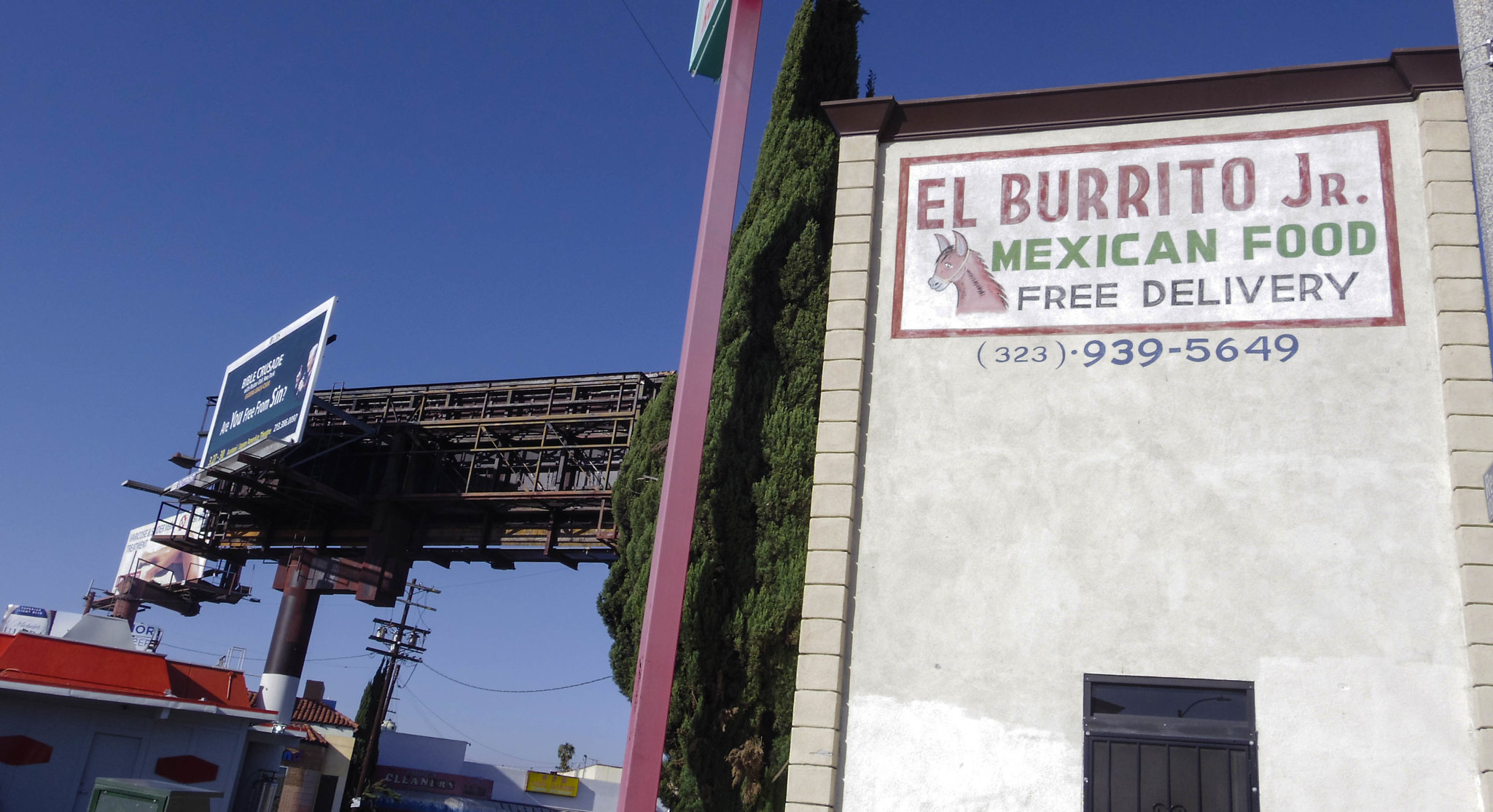This photo captures a bright, sunny day outdoors featuring a clear blue sky with no clouds. The central focus is a beige building on the right side of the image. Prominently displayed at the top is a rectangular sign with a red trim, inside which "El Burrito Jr." is painted in bold red letters. Directly below in green text, slightly offset to the right, it reads "Mexican Food." Underneath this, in black text, "Free Delivery" is inscribed. Below the sign in blue paint is the phone number, "323-939-5649." A brown donkey illustration accompanies the text. Adjacent to the building is a tall, dark green evergreen tree. The left side of the photograph showcases a vast expanse of clear blue sky. Further in the background, a large billboard or traffic sign can be seen, supported by a prominent beam, with a hint of another building featuring a red roof.